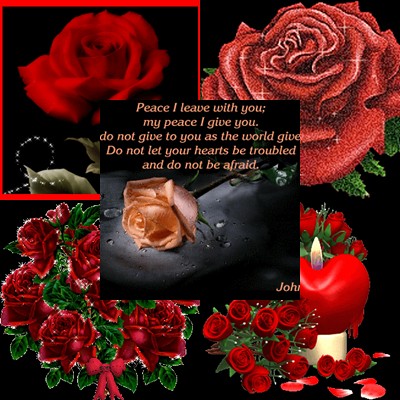This image features an artistic and digitally produced collage of four distinct rose-themed images arranged in a windowpane style format, with a central overlay featuring an inspirational text. The central text reads, "Peace I leave with you, my peace I give you. Do not give to you as the world give. Do not let your hearts be troubled and do not be afraid," in pink font against a black background. Each quadrant of the collage showcases different roses: the top left displays a dew-speckled cream-colored rose; the top right features a stylized, possibly plastic-looking red rose; the bottom left shows a bouquet of vibrant red roses intertwined with white lights; and the bottom right includes a heart-shaped lit candle surrounded by red roses. The overall color palette includes shades of red, black, white, green, tan, yellow, orange, gray, and off-white, contributing to the vivid and serene aesthetic of the artwork.